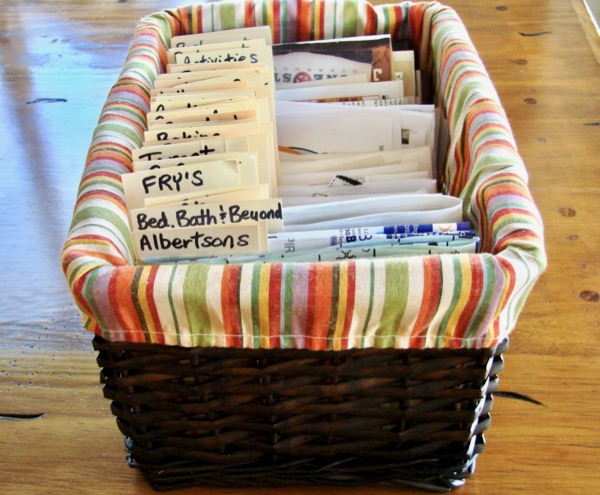The photograph captures a dark brown wooden basket placed on a glossy, light wood floor. The basket is lined with a multicolored fabric liner featuring stripes in hues of red, green, white, brown, orange, and purple. Inside the basket, numerous papers and documents are organized using a homemade divider system. The dividers are labeled with names such as Albertsons, Bed Bath & Beyond, Fry's, Target, and Activities, written in black on what appear to be sticky notes or pieces of paper. These documents seem to include bills, coupons, and perhaps receipts. The setup suggests a methodical approach to categorizing various household or personal paperwork.